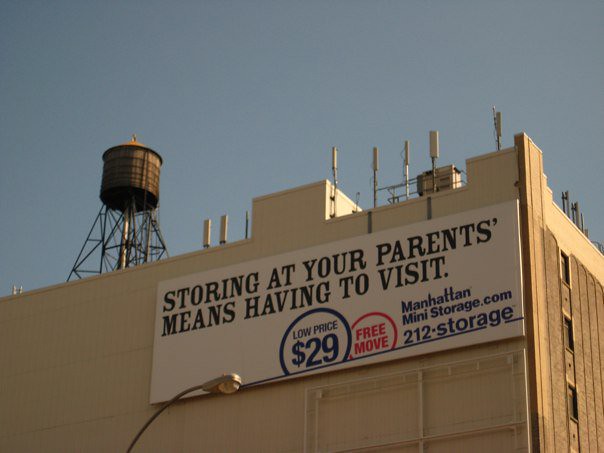The image captures an outdoor scene in landscape orientation, featuring the top portion of a three-story rectangular building bathed in yellow. The sky is a clear blue-gray, devoid of clouds, giving the photograph a crisp, unobstructed view. Taken from a low angle, the photo presents the building's corner on the right side, displaying three windows on each of its three visible stories. 

The majority of the image showcases the building's facade on the left. The structure has a predominantly flat roof, but the top left corner features a distinctive wire structure crowned with a cylindrical element, reminiscent of a water tower. A prominent white rectangular sign adorns the building's face, bearing black text that reads, "Storing at your parents means having to visit." Accompanying this message, a blue circle highlights a "Low price, $29," while a red circle advertises a "Free movie." Additional information in black lettering directs viewers to "manhattanministorage.com" and provides the phone number "212.storage."

In the lower section of the image, a streetlamp enters the frame from the bottom left, its pole bending to the right, with an oval lamp hanging down, contributing an urban touch to the scene.